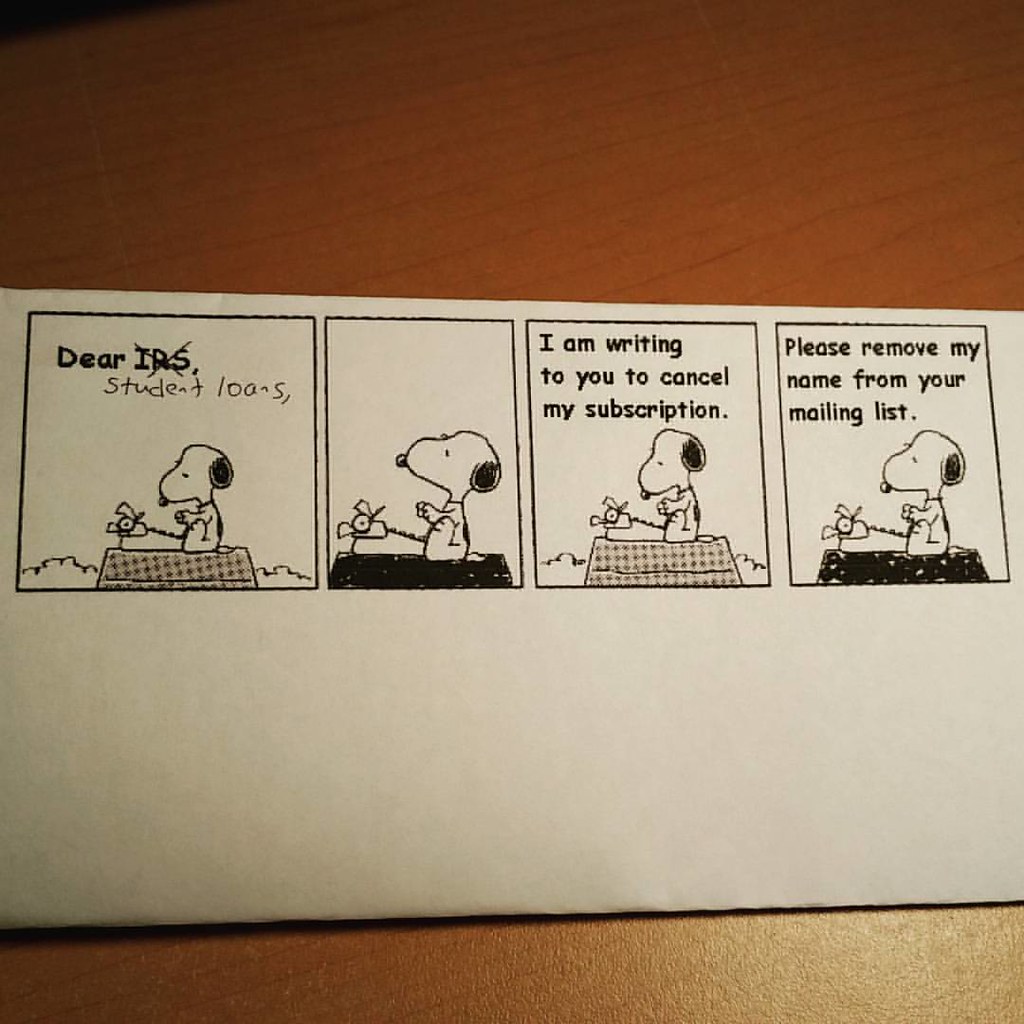This image captures a Peanuts comic strip featuring Snoopy, photographed on a light brown wooden table with a visible diagonal grain. The table is lightest at the bottom right corner and darker towards the top left, where part of the table's edge is visible. The square image shows a wide rectangular white paper, partially cropped on the left and right sides, possibly an envelope folded in half. The comic strip consists of four panels with black borders. The first panel is square, while the other three are taller rectangles, each depicting Snoopy sitting on his doghouse next to a typewriter. In the first panel, Snoopy types "Dear Student Loans," with the "IRS" text crossed out and replaced. The second panel shows Snoopy looking up thoughtfully. In the third panel, he types, "I am writing to you to cancel my subscription," and in the final panel, he continues, "Please remove my name from your mailing list."